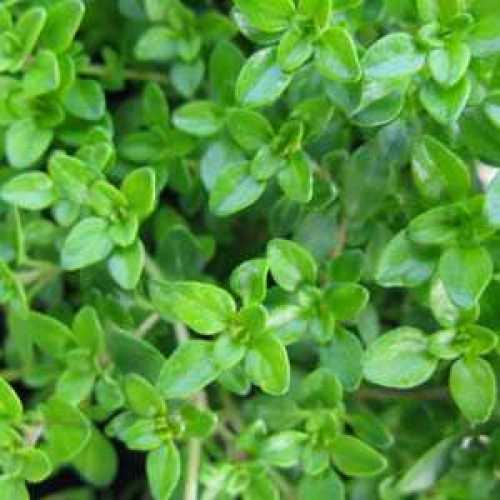The photograph captures a slightly grainy and blurry close-up of small, vibrant green leaves, arranged in dense bunches. These shiny leaves, each about an inch long and three-quarters of an inch wide, suggest the plant is very healthy and well-watered. The image, taken from a top view, reveals no flowers but rather clusters of tiny leaves, each resembling a small floweret with four or five petals. Lighter, somewhat faded stems can be seen in the background, interspersed with areas of black, adding contrast. The predominant colors are green and brown, with hints of gray and black primarily on the left-hand side of the image.